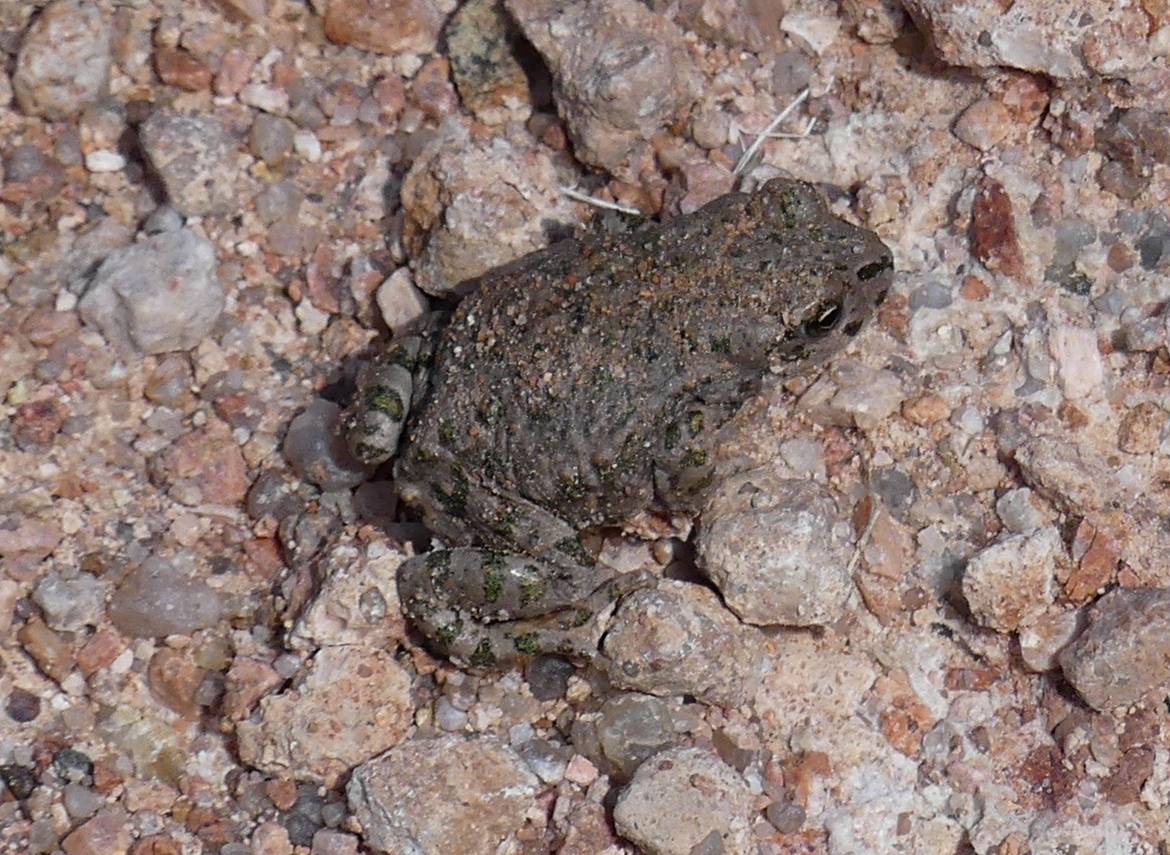The image depicts a small frog or toad, primarily grayish-brown in color with reflective dark green and black specks and markings, particularly prominent on its front and hind legs. Its skin appears a bit wet, and it has particles of sand and debris scattered across its back, giving it a camouflaged appearance. The frog is positioned amidst variously colored rocks—pinkish, gray, tan, and white—that resemble Himalayan pink salt with visible mineral deposits. The surface is a mixture of coarse sand and gravel. The frog is oriented so that its back legs are towards the left and its head towards the right, with its right eye visible. The overall setting suggests a dry, rocky habitat, potentially a desert-like environment or an exhibit in a zoo designed to mimic such conditions.